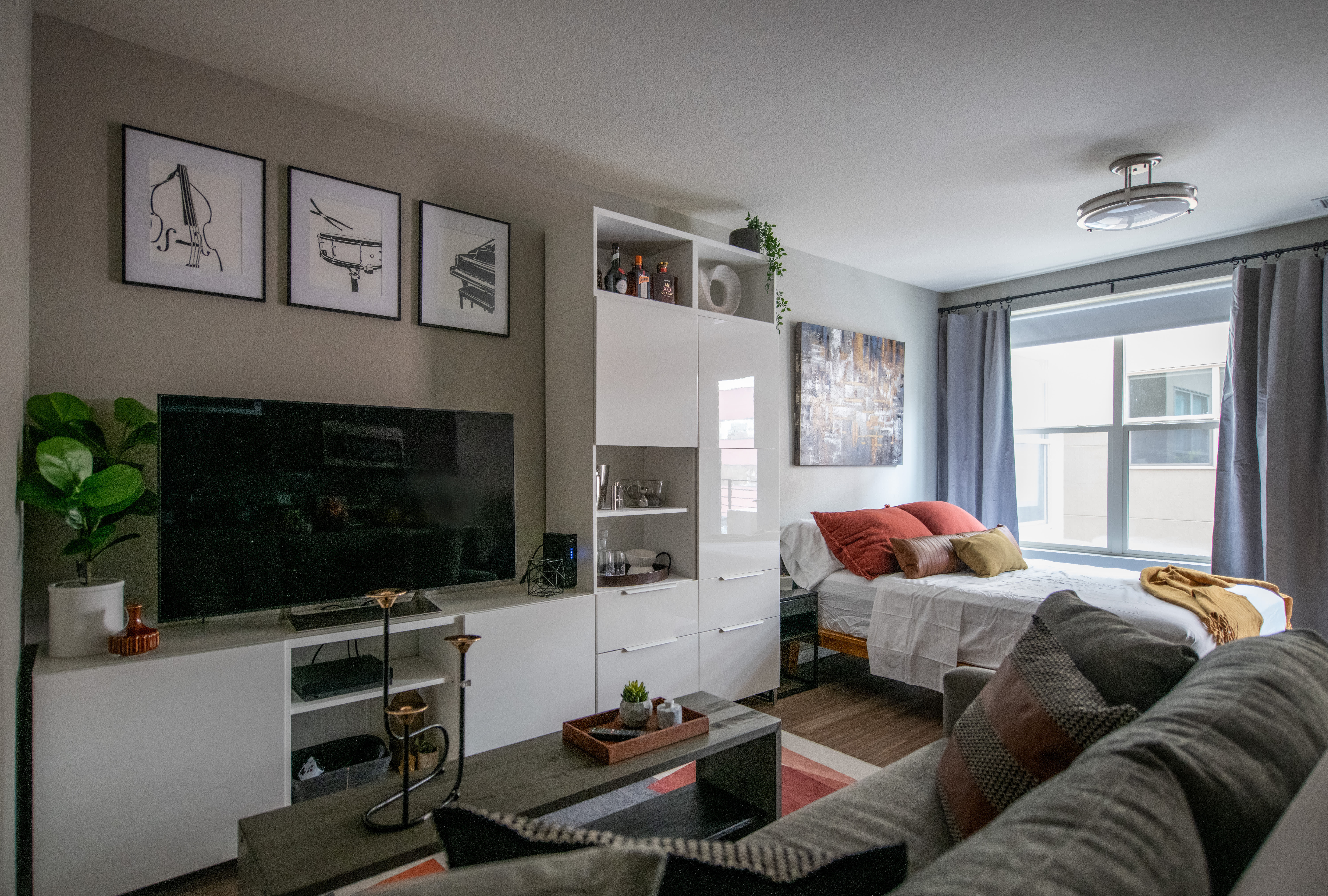The image depicts a cozy studio apartment that seamlessly integrates living and sleeping areas within a single rectangular space, wider than it is tall. Dominating the left side of the photo is a sleek entertainment setup featuring a large flat-screen TV mounted on white shelving units, which include multiple shelves and drawers. Adjacent to the TV is a verdant plant with lush green leaves, enhancing the homely atmosphere. Below the TV, a comfortable gray couch is positioned, adorned with throw blankets, opposite of which sits a thin, rectangular gray coffee table. 

The right side of the room houses a neatly made bed adorned with white bedding, accented by rust and tan pillows, and a gold throw blanket. Above the bed hangs a large piece of artwork, contributing to the room's aesthetic appeal. A round ceiling light is installed near the bed, providing a warm ambiance. Drawing attention to the wall space, three framed pictures of musical instruments are positioned above the TV area.

The room also features a sizable window with blue blinds drawn open, offering a direct view of a neighboring apartment's window, suggesting the apartment resides in a high-rise building. The tan-colored walls add a subtle warmth to the space, complementing the overall neutral palette of grays and whites.

In essence, the apartment presents a well-organized and inviting environment that combines functional living and sleeping quarters, with a distinct homey charm that's reminiscent of a cozy hotel suite.